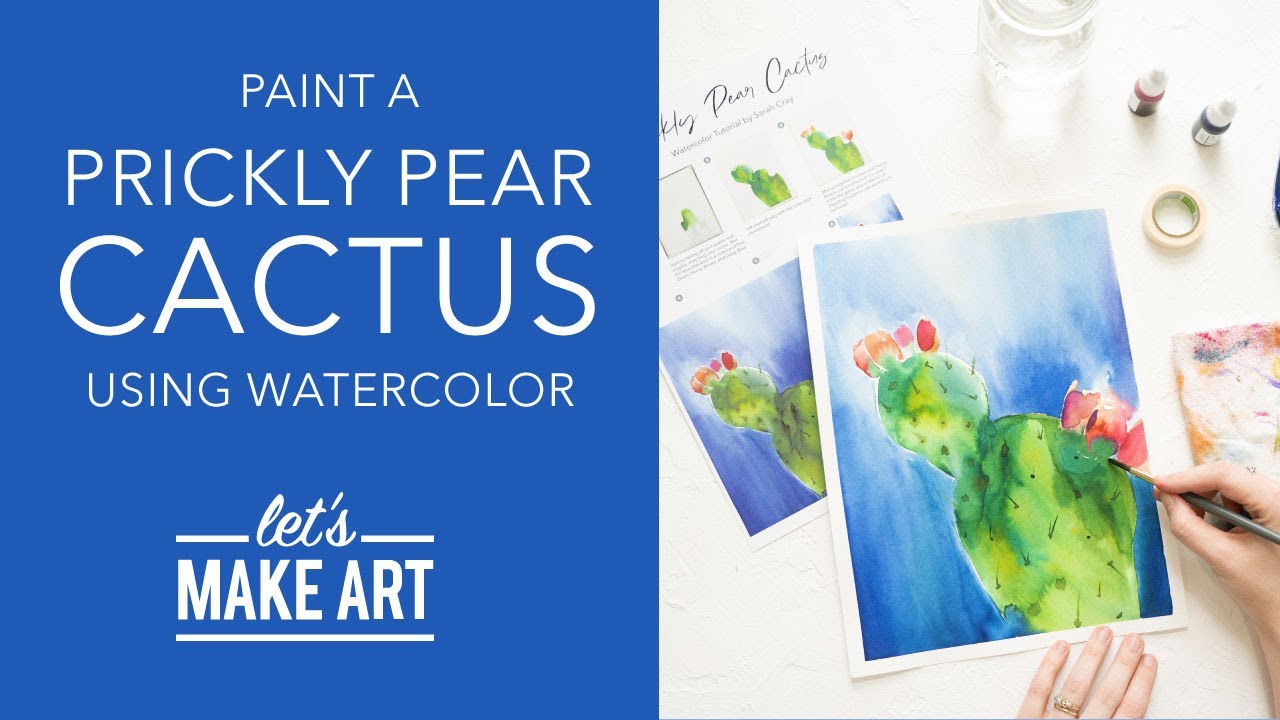The image appears to be an advertisement or flyer for an art class or product focused on painting a prickly pear cactus using watercolors. The layout is divided into two halves. The left half features a bright cobalt blue background with white text that reads "PAINT A PRICKLY PEAR CACTUS USING WATERCOLOR," and a logo at the bottom that says "let's make art" with the word "let's" in cursive. On the right half, there is a detailed real-life scene of a person actively painting a prickly pear cactus. The person, identifiable by their feminine hands and a wedding ring on their left hand, holds a paintbrush in their right hand. The painting in progress is green with protruding parts and vibrant pink, orange, and red flowers, set against a blue and white background. Various art supplies are visible on the white table: jars of liquid watercolor, a container of water, a roll of tape, and a paper towel with paint marks. There’s also an instructional printout that outlines the steps to paint the prickly pear cactus, serving as a guide for the artist. This comprehensive setup suggests that the image is promoting a structured and detailed approach to watercolor painting.